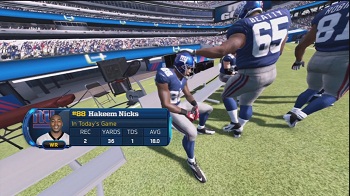This image appears to be a hyper-realistic screenshot from an American football computer game, captured in low resolution. It features players near the sideline of a stadium, with a focus on one player seated on a bench wearing a dark blue jersey, gray pants, and a helmet displaying "NY" in white. This player is being patted on the helmet by a larger teammate. The players' uniforms include distinct red stripes down the sides of their trousers, white numbers on their jerseys, with one player displaying the number 65 and the name "Beatty" above it. 

The backdrop includes a crowded stadium with multilevel seating sections, filled with attendees. The grass and surrounding textures give an impression of a realistic football field, though closer inspection reveals the pixelated, digital nature indicative of a video game environment. 

On the left front of the image, an infographic overlay features a head-and-shoulders portrait of a player named Hakeem Nix, with statistical numbers listed below, although these details are too small to read clearly. The words "today's game" are visible in yellow on the graphic, adding to the in-game broadcast feel. The entire composition strongly mimics the atmosphere and visual elements of a real-life American football game, despite its digital origins.